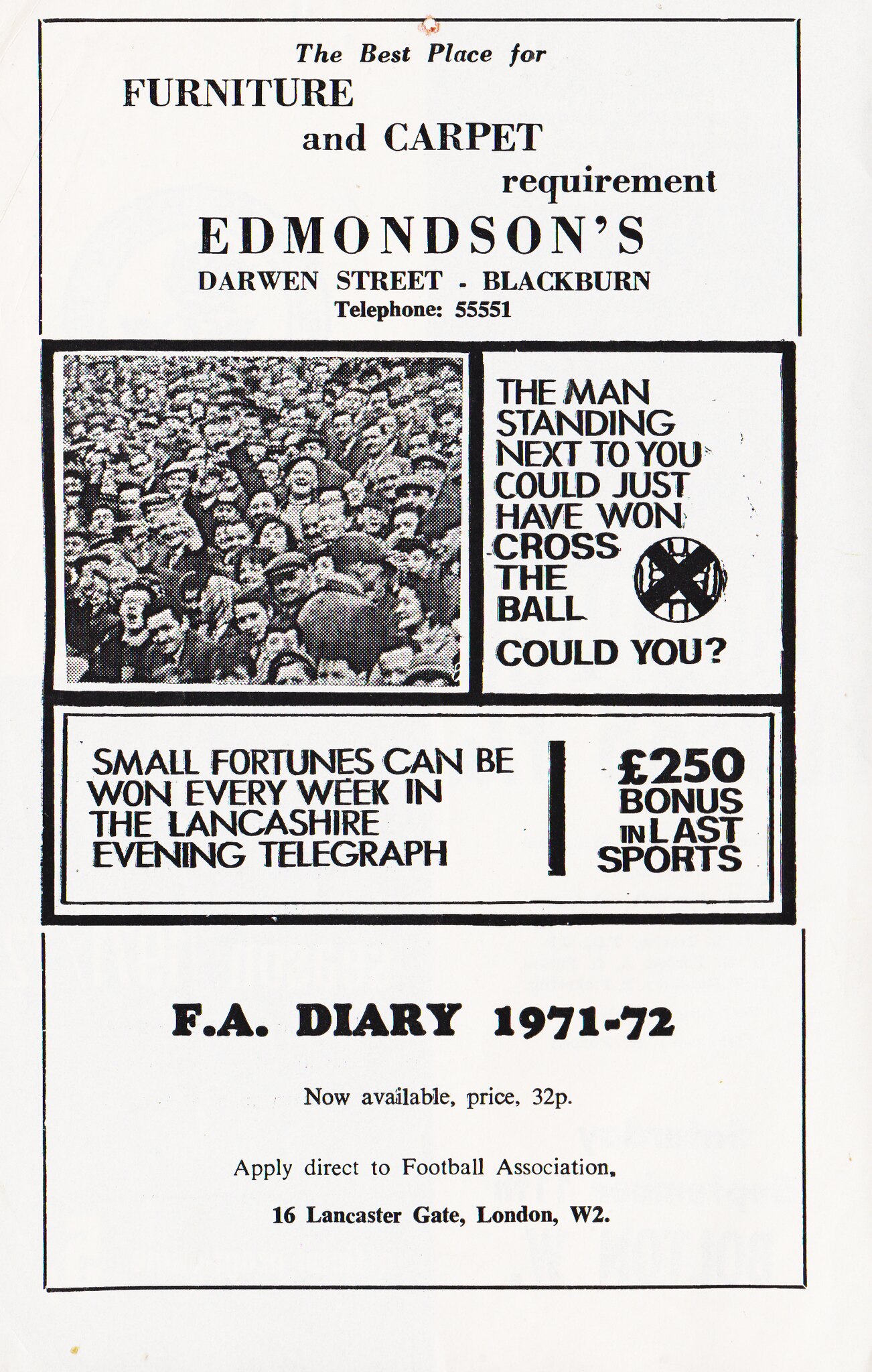The image depicts a black-and-white page from a sporting manual or magazine. At the top, an advertisement promotes Edmondson's as "The Best Place for Furniture and Carpet Requirements," located at Darwin Street, Blackburn, with the telephone number 55551. Central to the image is a photograph of a cheering crowd, featuring men in black hats and women dressed up. To the right of the photo, there's text suggesting a contest: "The man standing next to you could just have won 'Cross the Ball.' Could you?" Below this, another section reads: "Small fortunes can be won every week in the Lancashire Evening Telegraph. £250 bonus in last sports." At the bottom, it announces, "F.A. Diary 1971–72 now available, price 32p. Apply direct to Football Association, 16 Lancaster Gate, London W2."